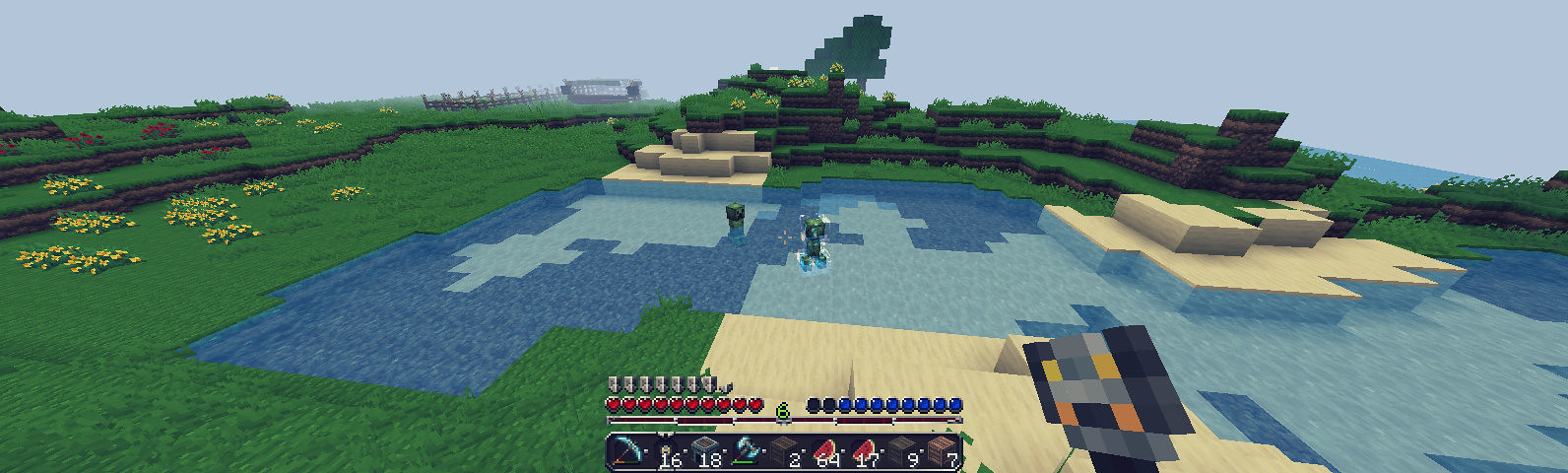This screenshot from the pixelated video game Minecraft captures a detailed outdoor scene. The main focus is a character holding a lantern torch in their right hand. They're standing by a body of water, where a Creeper lurks. The environment features a lush grassy area to the left adorned with red and yellow flowers, as well as a few scattered trees. A beachy zone borders the water, transitioning into what looks like either sand or a type of brick. In the distance, on the left horizon, a structure can be seen. The game's interface shows a panel at the bottom displaying the character's inventory with items like a pickaxe, watermelon, crates, and other resources. The character appears to have full health. Overall, this scene is a vibrant mix of natural elements and pixel-art charm, characteristic of Minecraft's block-style graphics.